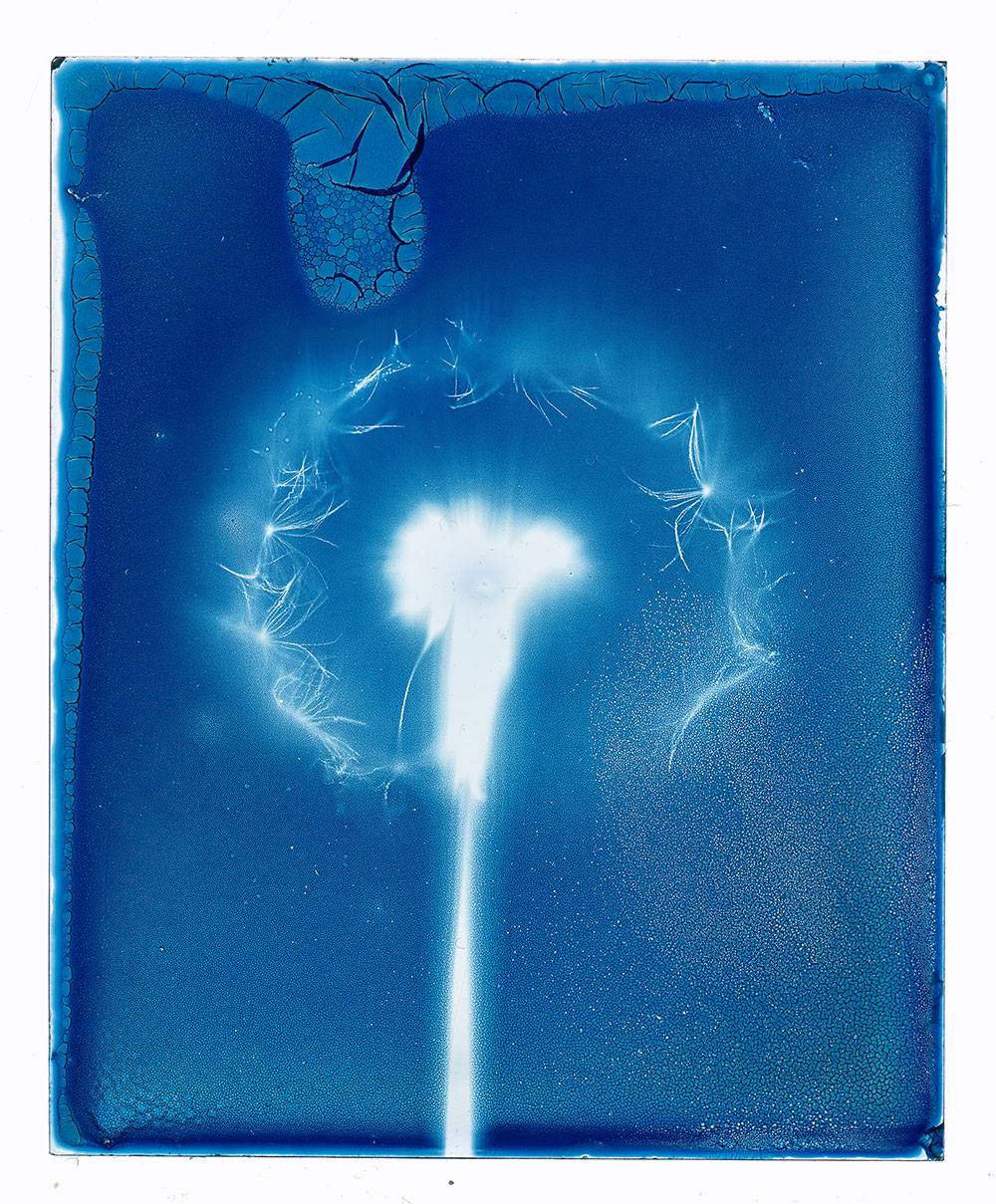The image depicts a striking, deep royal blue background, which appears to be a textured, ridged surface similar to a crusty bluish clay or glass. At the center of this vivid blue canvas is a captivating, bright white light shaped like a flower, extending down into what resembles a stem. The flower-like form is central to the composition, surrounded by intricate, stringy white lines that evoke the appearance of electricity or a delicate dandelion’s petals in printmaking. Tiny white sparks glitter around this central motif in a circular arrangement. The overall effect is one of an artistic cyanotype, featuring only shades of blue and white, blending natural floral imagery with a surreal, almost otherworldly light display, accentuated by bubbly marks in the bottom right-hand corner. This evocative piece leaves a sense of wonder about the material and artistic techniques employed to create such an engaging visual experience.